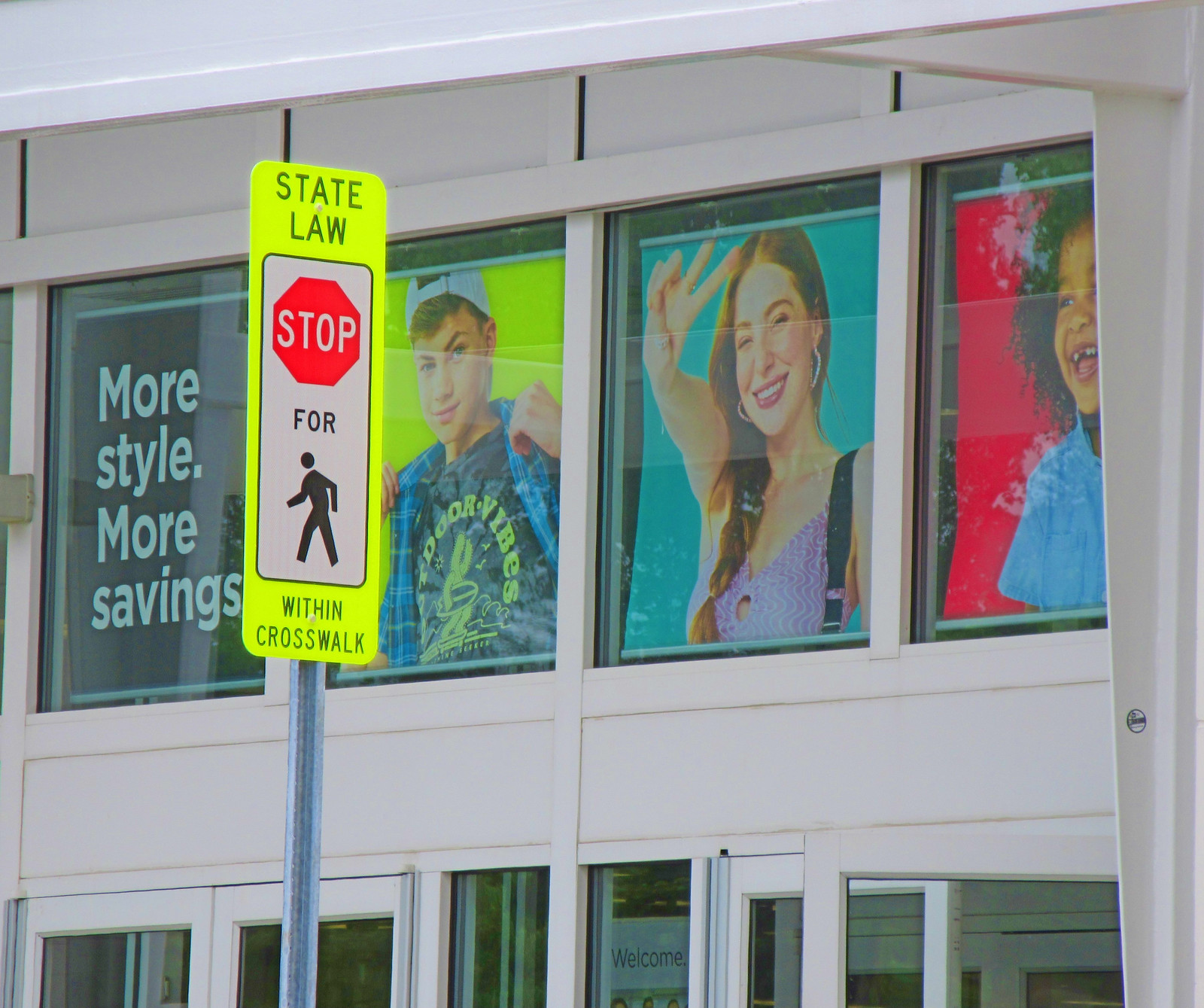This photograph features a two-story building with its first floor partially visible, revealing the tops of windows and the corner of an opening door. The second story prominently displays several large advertisements in the storefront windows. One advertisement, set against a green backdrop, reads "More Style, More Savings" in white letters. Another advertisement showcases a young boy with a backpack and a white hat. To the right, a girl with brown hair poses with a peace sign while wearing a purple shirt. Another child with curly dark hair, wearing a blue t-shirt, stands out against a vivid red background. In front of the building, a bright yellow neon road sign commands attention, stating "State Law: Stop for" followed by a pedestrian walking symbol, with "Within Crosswalk" written in black letters.